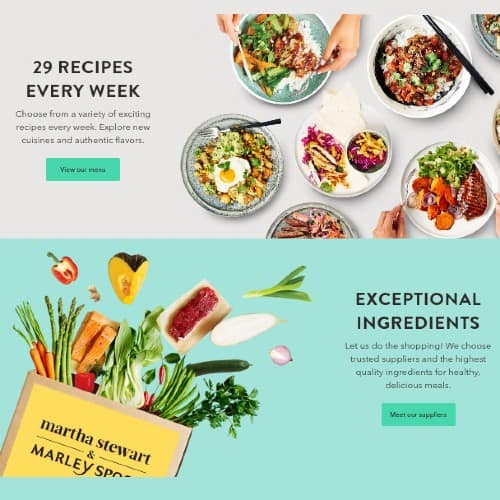This vibrant landing page features an array of enticing food images and informative text. On the right, several dishes are showcased alongside a person's hands. Starting from the top, there is a dish with eggs, croutons, and salad fixings. Below that is a plate filled with red and brown meat, rice, and vegetables, with a hand hovering over it. Adjacent to this, a white bowl contains more meat and vegetables mixed with a red and orange sauce atop white rice.

Further down, a delicious-looking fajita with grilled chicken, cut peppers, and caramelized onions is displayed. To the right, another hand is seen next to a plate of sweet potatoes, grilled salmon, and mixed greens. 

On the left-hand side of the page, a bold black header states "29 recipes every week," followed by a lighter black text description: "Choose from a variety of exciting recipes every week. Explore new cuisines and authentic flavors." Below this text is a rectangular teal button with dark green text that reads "View Our Menu."

Towards the bottom of the page, a light blue section showcases various fresh ingredients like peppers, carrots, okra, bread, lettuce, and some kind of cut fruit, emerging from a brown bag. The bag features a yellow label with black text that reads "Martha Stewart and Marley," partially cut off with "SPO" visible.

On the right side, bold text proclaims "Exceptional Ingredients." Below, standard black text explains, "Let us do the shopping. We choose trusted suppliers and the highest quality of ingredients for healthy delicious meals." Another teal rectangle with dark blue text instructs visitors to "Meet Our Suppliers."